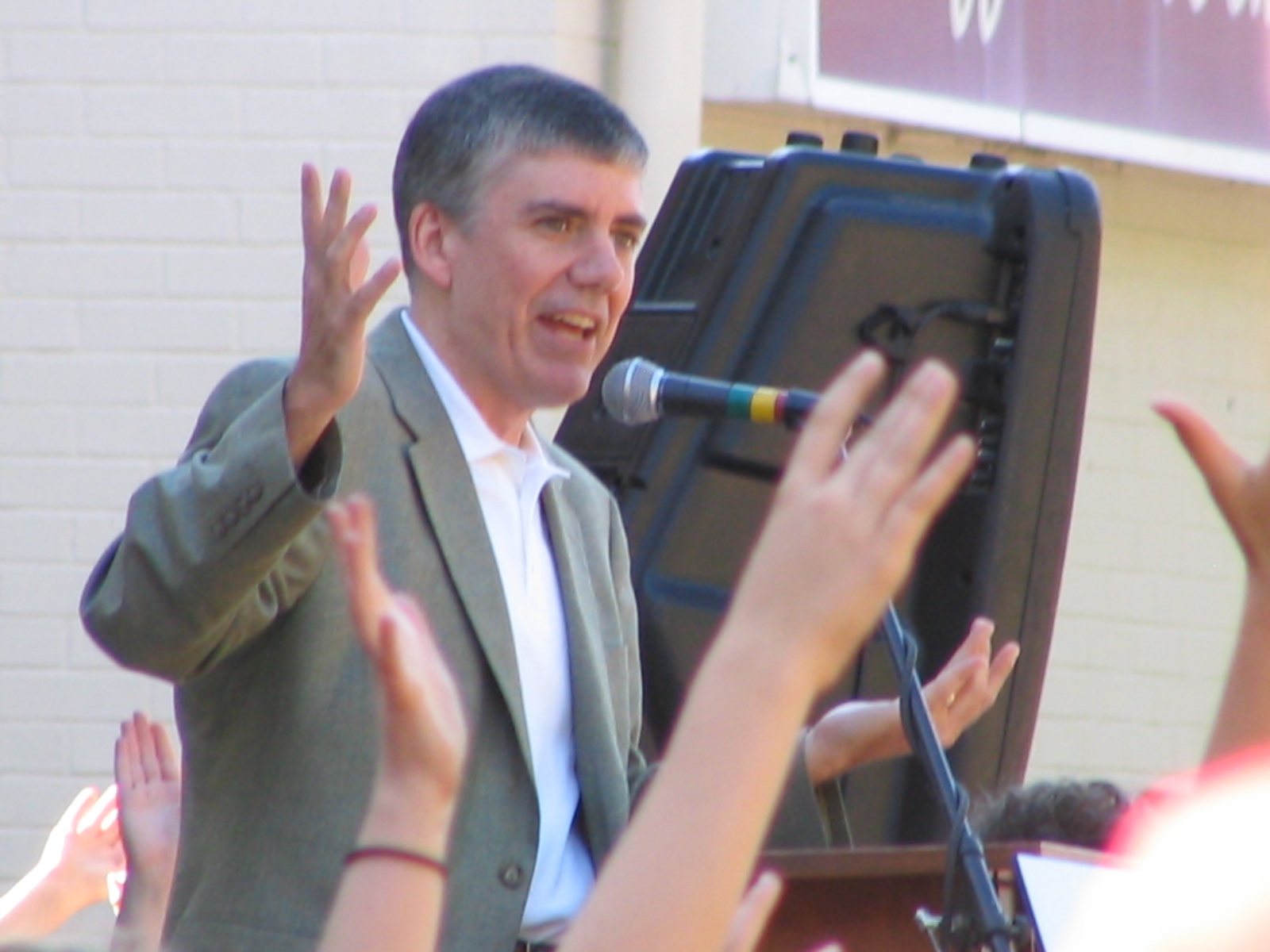In this photograph, a man, appearing to be between 40 and 45 years old, is standing behind a podium with a microphone wrapped with green, yellow, and red bands, suggesting he is giving a speech, presentation, or even a sermon. The background features the off-white, cream-colored exterior of a building, indicating an outdoor setting bathed in natural sunlight. To the right, there's a large black PA speaker on a stand, and a reddish sign with a white outline is visible in the top right corner. The man has short, dark gray hair with lighter gray accents, and wears an open gray blazer over a white button-down shirt or possibly a polo shirt. He is gesturing with both arms raised, and his intent expression suggests he is passionately engaging with his audience. The crowd in front of him is visibly involved, with several hands and wrists raised towards him, contributing to the dynamic atmosphere of the scene.